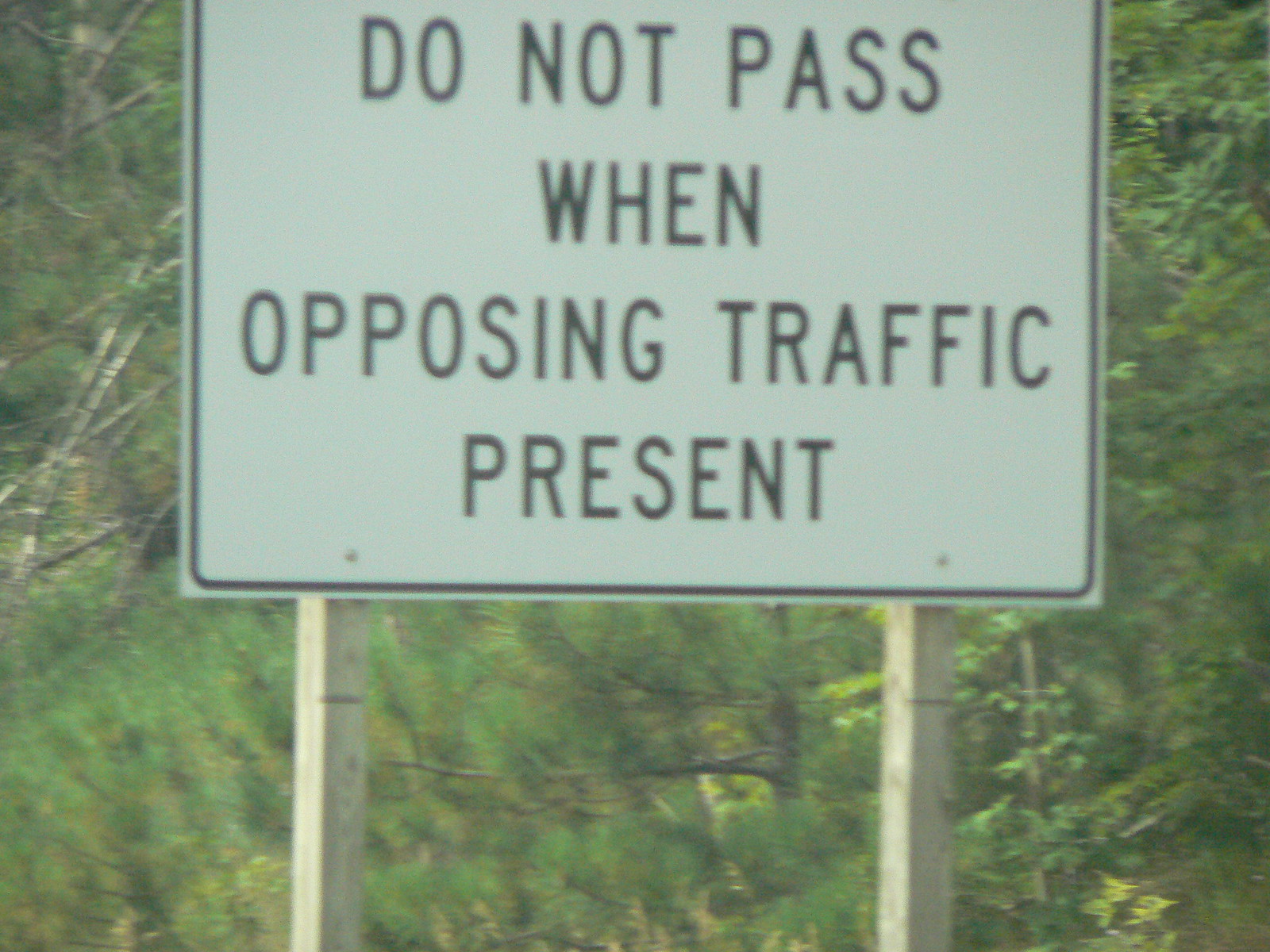**Caption:**

A detailed close-up of a white road sign attached to two square wooden poles, which are positioned at the back left and right of the sign, respectively. The sign features a thin black border and bears the message "DO NOT PASS WHEN OPPOSING TRAFFIC PRESENT" in bold, black letters. The background is densely packed with vibrant green leaves and branches from surrounding trees, creating a lush, natural backdrop. Some bare branches appear towards the right side of the image, and the trunk of a tree is visible near the center of the frame, partially obscuring the sign. The photograph has a somewhat grainy texture and lacks vividness, giving it a rustic and subdued appearance.